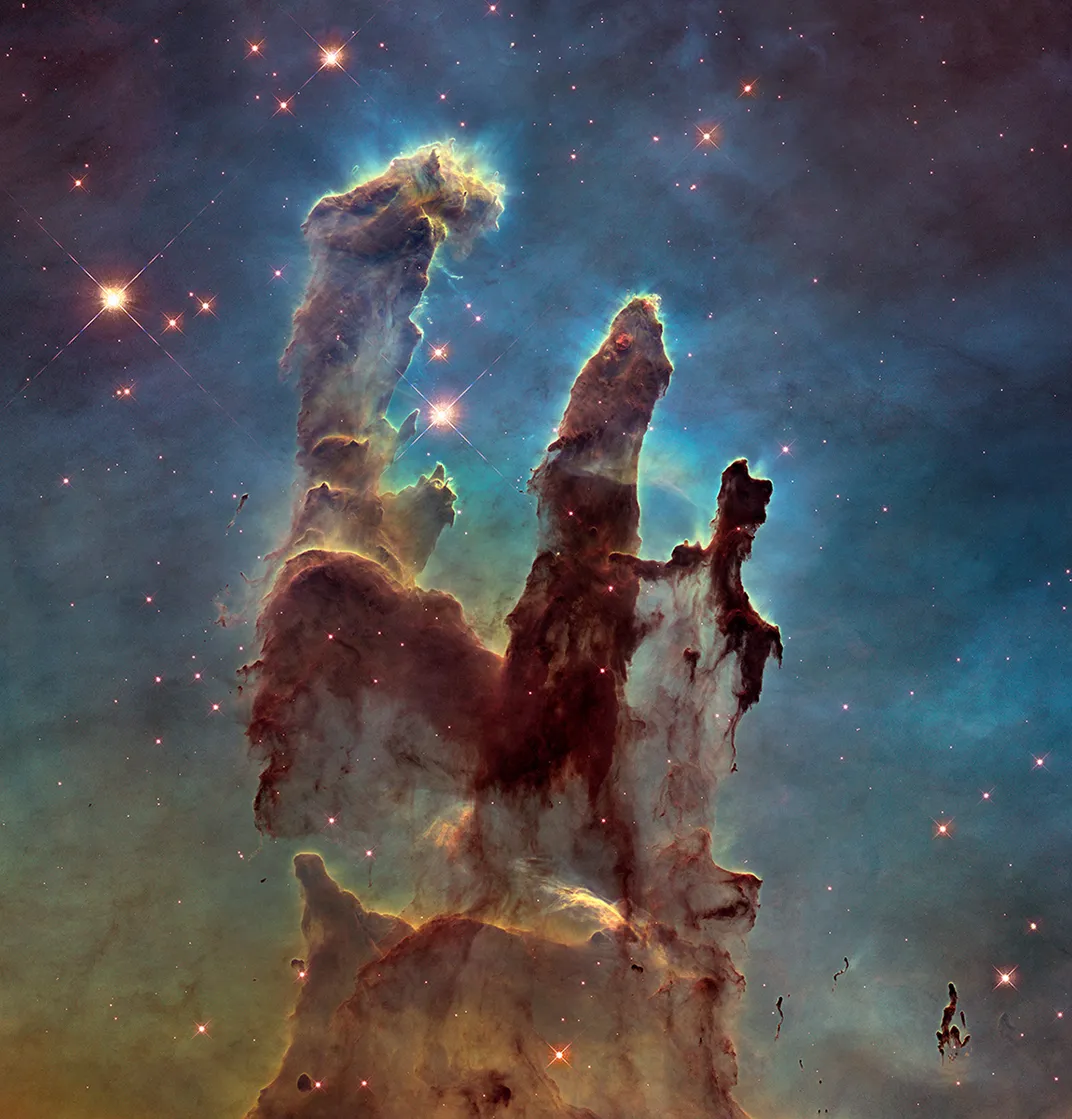This image from space, likely taken by the Hubble Telescope, captures the majestic Pillars of Creation within a nebula. The starscape forms a stunning backdrop, featuring numerous bright, shining stars with four-pronged cross-shaped artifacts caused by the telescope. The scene is dominated by towering, cloud-like pillars of gas and dust, which appear to burst upward from the bottom. These spectral pillars display a range of colors, from deep reds and browns to light blues and oranges, giving them a ghostly, almost translucent appearance. The leftmost pillar is particularly tall and prominent, with two other significant formations, one of which has an offshoot to the right. This celestial landscape is both awe-inspiring and intricate, combining the dark vastness of space with the vivid, rich hues of the nebula's gas clouds.